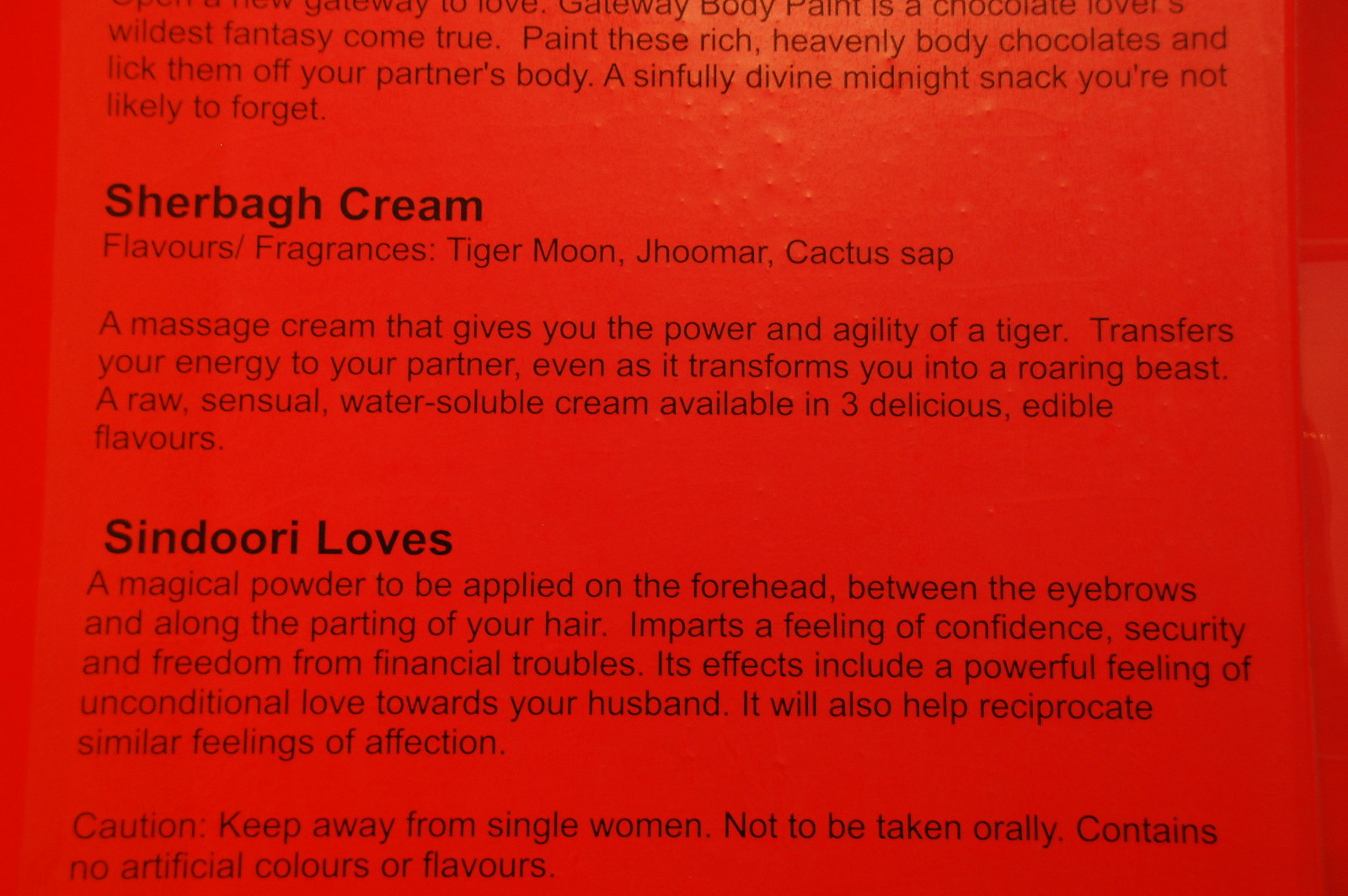The image depicts the back label of a product, set against a red backdrop with black text. At the top, the label describes Gateway Body Paint as "a chocolate lover's wildest fantasy come true." It suggests painting these rich, heavenly body chocolates on a partner and enjoying a sinfully divine midnight snack. Below this, there is information about various sensual products:

1. **Sherba Cream**: This is a massage cream available in three flavors and fragrances – Tiger Moon, Jumar, and Cactus Sap. It's described as a raw, sensual, water-soluble cream that gives the user "the power and agility of a tiger," transferring energy to the partner and transforming the user into a "roaring beast."

2. **Sindori Loves**: This is a magical powder meant to be applied on the forehead between the eyebrows and along the parting of the hair. It imparts a feeling of confidence, security, and freedom from financial troubles, enhancing unconditional love towards one's husband and reciprocating similar feelings of affection. It also includes a caution to keep away from single women and is not to be taken orally.

Overall, the label combines vivid descriptions of exotic, intimate products with bold claims of their transformative effects, all presented with black text over a striking red background.